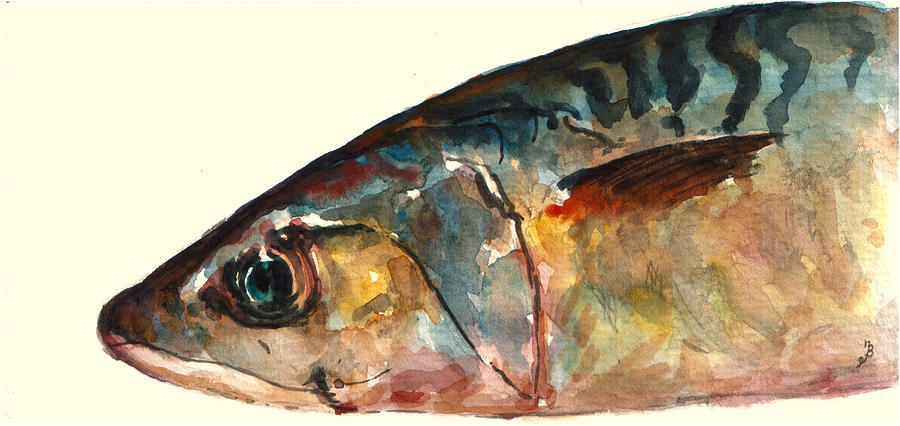This watercolor painting depicts a fish viewed from the head to its midpoint, lying on its side against a light pale yellow background. The fish’s left profile is showcased, with a small face widening towards the body. The back of the fish features a blend of blue tones with darker zigzagged stripes, while the top exhibits dull shades of grey and brown. A single fin, brown with black accents, sticks straight out from the body. The fish’s eye is a dark blue with a glassy appearance and black accents, and its mouth remains closed. Red hues surround the gills, giving way to a multicolored lower body adorned with pinks, salmon shades, gold, and off-green tints. Striking vertical black stripes extend from the back to just about where the fin protrudes. The intricate blending of colors and detailed textures yield a vivid portrayal of underwater life.